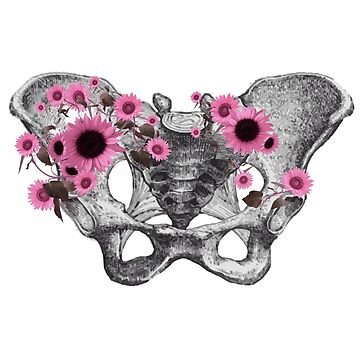This detailed black-and-white artwork depicts an anatomically accurate drawing of a human pelvis, shaded skillfully with what appears to be pen or pencil. The pelvis is positioned centrally and includes a portion of the spine. Surrounding the top part of the pelvis are vibrant illustrations of pink sunflowers in full bloom, featuring roughly 30 small petals each. The flowers vary in size and are more concentrated on the top left side, with an approximate total of 15 scattered across the pelvis. The sunflower petals range from light to medium pink, while the centers vary from dark pink to dark brown. The background remains stark white, emphasizing the intricate bone structure and the contrasting colorful blooms, creating a visually striking piece of art.